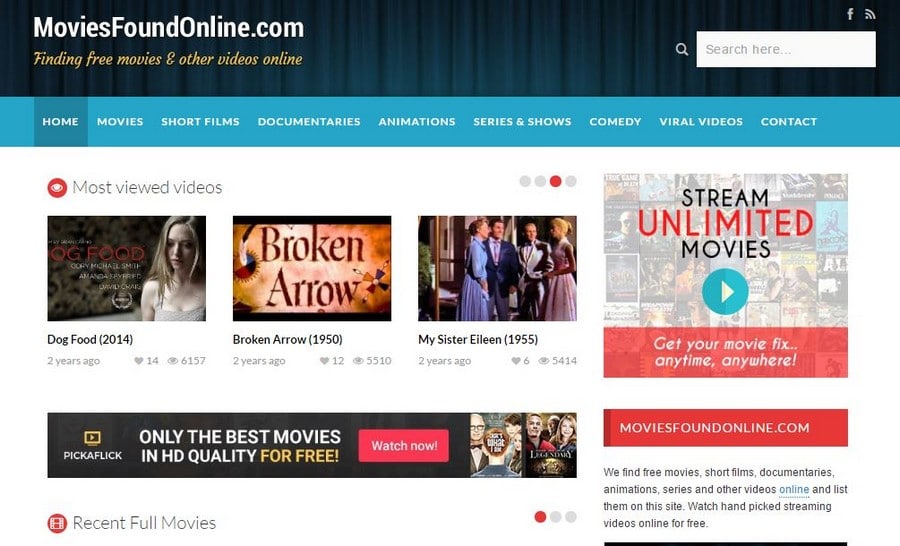This image is a detailed screenshot of the website MoviesFoundOnline.com. At the very top, there's a banner resembling a classic movie curtain. Below the banner, the website's name is prominently displayed as "MoviesFoundOnline.com" with the tagline "Finding free movies and other videos online" underneath. On the right side of this section, there’s a search bar labeled "search here" alongside both a Facebook icon and a Wi-Fi symbol.

Directly below this is a blue navigation menu with several options: "Home" (which is highlighted), "Movies," "Short Films," "Documentaries," "Animations," "Series and Shows," "Comedy," "Viral Videos," and "Contact." 

Further down the page, there is a section titled "Most Viewed Videos," showcasing small thumbnail images of three movies: "Dog Food" (2014), "Broken Arrow" (1950), and "My Sister Eileen" (1955). Each of these thumbnails shows that they were last watched two years ago.

Adjacent to this, there is an advertisement box promoting "Pick a Flick," which touts "only the best movies in HD quality for free," with a call-to-action button "Watch Now." Below the ad, there is a section labeled "Recent Full Movies."

On the right side of the page, another advertisement encourages visitors to "Stream unlimited movies" with a slogan "Get your movie fix anytime, anywhere." At the very bottom, the website's name is reiterated in a red box as "MoviesFoundOnline.com."